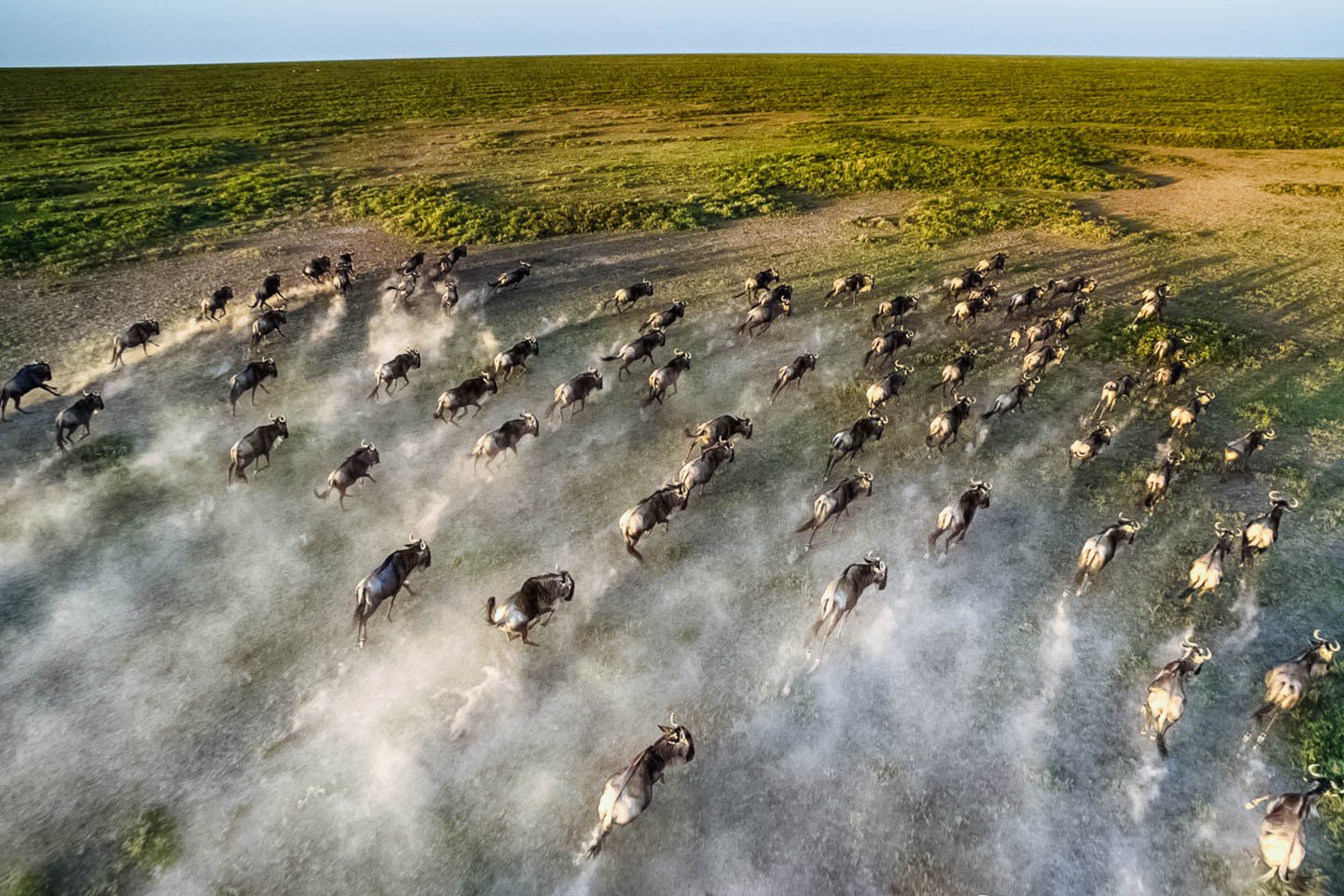The photograph captures an overhead view, possibly taken from a drone or helicopter, of a large herd of approximately 40 wildebeest stampeding across the African landscape. The animals, identifiable by their distinct curved horns, are running in a slightly spread-out but cohesive wedge formation, with the forefront of the group more densely packed than the rear. They traverse a mostly flat terrain characterized by patches of scrub brush and a mix of yellows and beiges, indicating less well-watered areas. The ground beneath their hooves is heavily trampled, contrasting with the more vegetated surroundings outside their path. A massive cloud of dust rises behind them, accentuating their rapid movement. In the distance, the horizon features clear blue skies, highlighting the dynamic energy of this captivating scene.